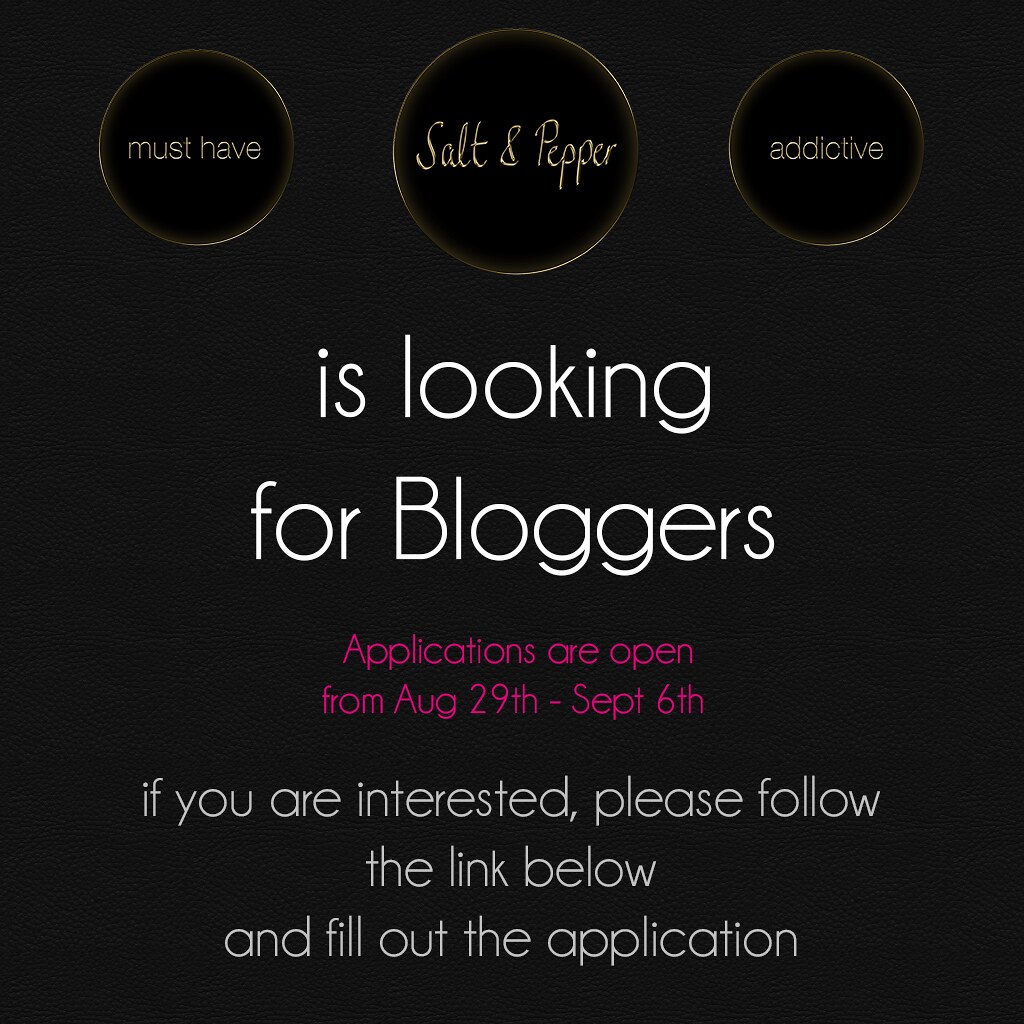The advertisement for the blog "Salt and Pepper" is set against a solid black background. Dominating the center, the text prominently reads in bold white lettering: "Salt and Pepper is looking for bloggers." The text "Salt and Pepper" appears to be designed as the blog's logo, potentially in a distinct cursive or stylized font. Below, vivid pink-red text announces "Applications are open from August 29th through September 6th." Following this, a slightly subdued white text directs interested applicants to follow a link to fill out an application, although the actual link is not visible. Above this main text block, three small circles with golden yellow outlines feature the phrases "must have," "Salt and Pepper" (matching the blog's logo style), and "addictive," adding an additional layer of emphasis. The varying colors, fonts, and the structured sequence of information make it a visually engaging call for bloggers, all set against a plain black backdrop to enhance readability and focus.